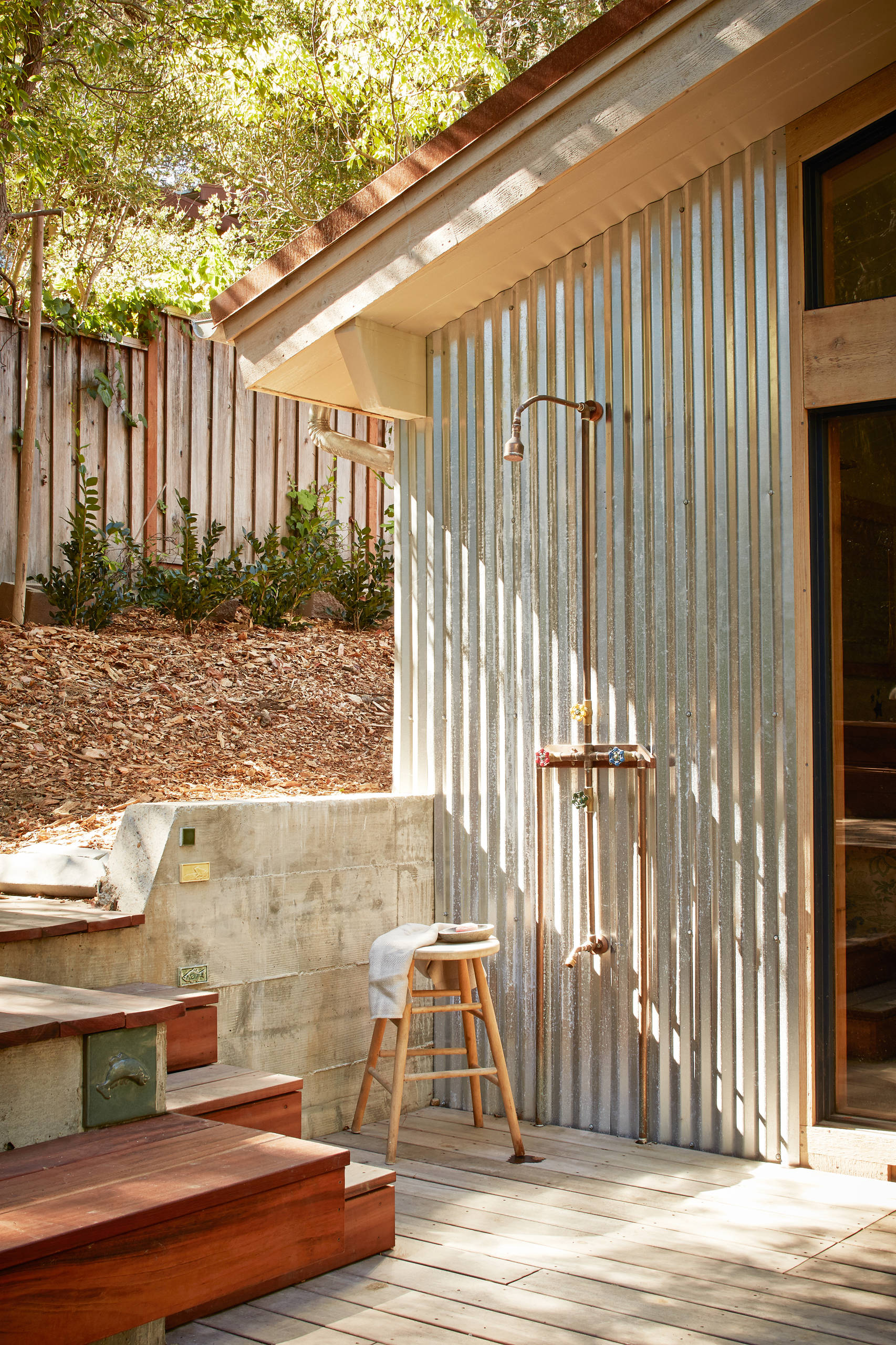This color photograph captures a serene backyard patio scene in the summer, featuring the left side of a corrugated silver metal house accented with gold and copper lines. Prominent in the image is an outdoor shower with copper pipes and fixtures. The shower setup includes a brass shower head spraying water, a middle faucet, and a small faucet at the bottom for washing feet. Next to the shower, there is a small wooden bench with a bar of soap, a ceramic cup, and a towel draped over it. The area is bordered by a sturdy concrete retaining wall adorned with plaques. In front of the wall, the ground is covered with dried leaves and mulch. There are also some leafy plants and green bushes growing against a tall wooden fence. Dark wooden steps, adorned with a brass fish, lead up toward the bottom left corner of the image. In the background, tall leafy trees are visible, adding to the lush, natural ambiance of the photograph. There are no people or animals in this vertically oriented image.